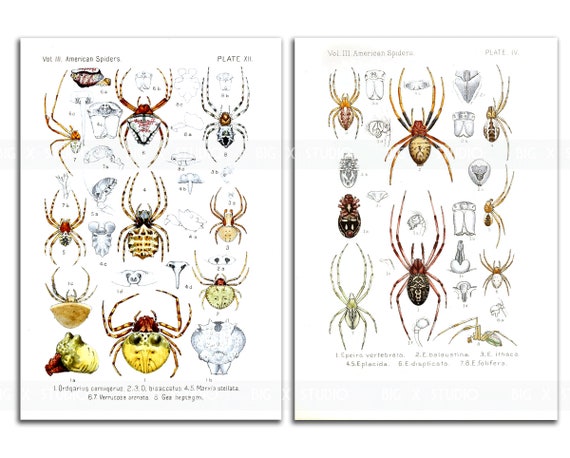The image is divided into two pages that resemble book illustrations, titled "Volume 13, American Spiders" on the left and "Volume 3, American Spiders" on the right. Each page shows a collection of spiders in various sizes, colors, and forms. The left page is labeled "Plate XII" and features around eight or nine spiders, including a notable yellow spider with giant legs and a red and black spider, depicted with detailed anatomical parts labeled and separated. The right page, labeled "Plate IV," displays seven spiders, with two significantly larger red-colored spiders in the middle, surrounded by a mix of other species and anatomical drawings. Both pages include the scientific names of each spider at the bottom, though some are difficult to pronounce. The spiders are shown in rows and columns, showcasing an array of body and leg lengths, and some are illustrated in partial views, capturing different angles and profiles.